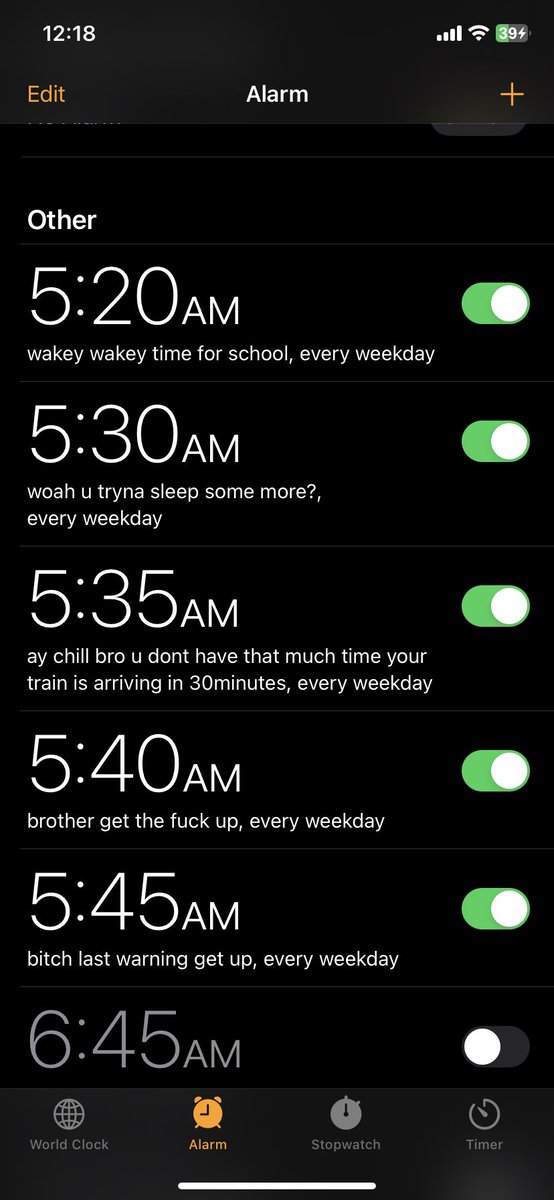The screenshot taken from a phone displays a black background with several details visible. The top of the screen shows the current time as 12:18 AM, along with an indication of four bars of cellular signal, a Wi-Fi logo, and a battery level at 39%. In an orange font, the word "EDIT" is displayed, and in white, the word "ALARM" is present. Additionally, there is an orange plus symbol.

Below these elements, the screen lists various alarms. The first section labeled "OTHER" includes detailed information with times and corresponding toggle bars. Here is the breakdown:

1. At 5:20 AM, the text reads "wakey-wakey time for school every weekday." The toggle is green, indicating the alarm is set.
2. At 5:30 AM, the text reads "whoa, you trying to sleep some more every weekday." The toggle is also green.
3. At 5:35 AM, the text reads "hey chill bro, you don't have that much time, your train is arriving in 30 minutes every weekday." The toggle is green.
4. At 5:40 AM, the text reads "brother, get the fuck up every weekday." The toggle is green.
5. At 5:45 AM, the text reads "bitch, last warning, get up every weekday." The toggle is green.

The final entry shows an alarm set for 5:20 AM with the text "OTHER," but this toggle is gray, indicating that this alarm is turned off. 

Overall, the screenshot captures a series of meticulously scheduled alarms, each with a unique, humorous message emphasizing urgency as the morning progresses.